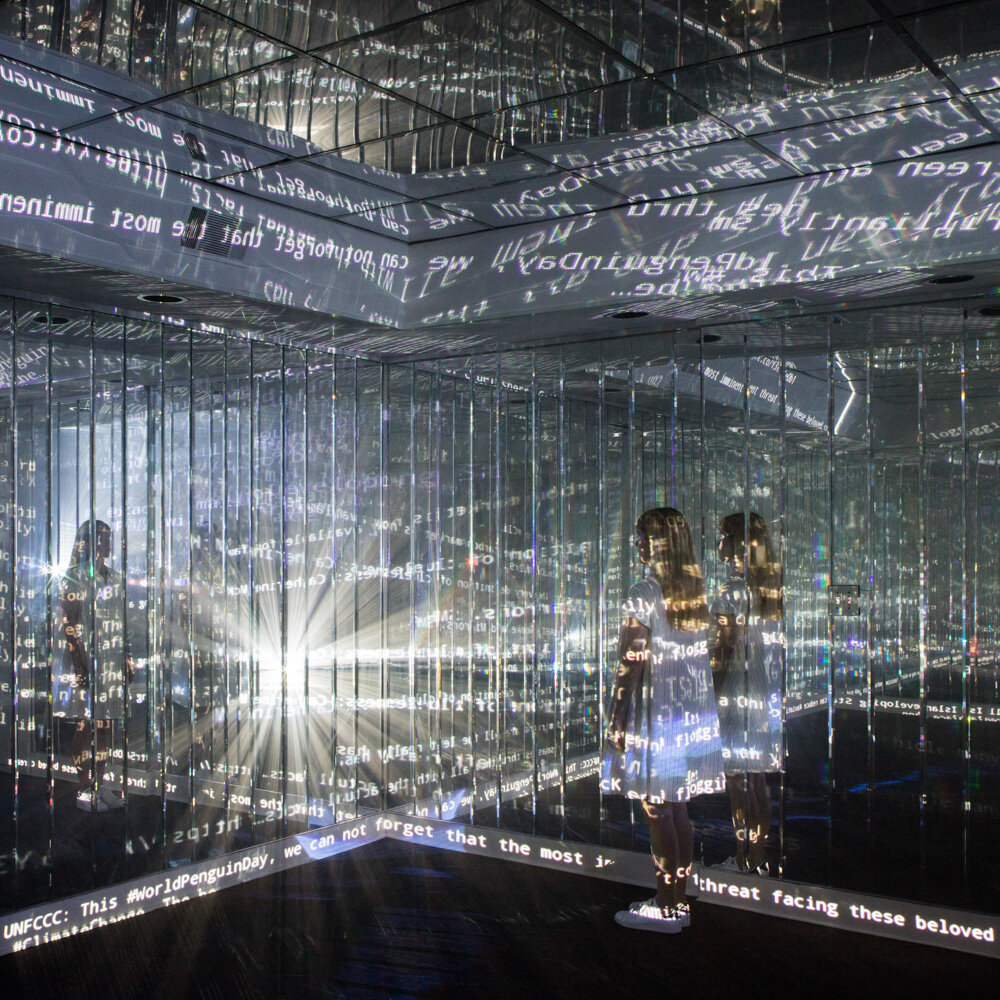A young blonde woman is standing in the corner of a sophisticated art installation, which appears to be an elaborate room full of thin mirror panels. Positioned on the right side of the image, she looks diagonally to the left, where intense, almost sunlight-like reflections are emanating from. The room's walls are adorned with narrow mirror slats, approximately six inches wide, extending nearly from floor to ceiling and interspersed with silver vertical bars. The ceiling is similarly mirrored, featuring square black strips separating glass panels. Text is projected onto the baseboard trim and reflected across the entire space, creating an intriguing visual echo. The mirrored surfaces scatter the text in every direction, enhancing the illusionary effect. The fragmented words include phrases like "This World Penguin Day, We Cannot Forget That The Most" and "Threat Facing These Beloved," although some remain unreadable due to the reflections. The floor is dark brown, adding to the contrast. The woman herself wears a short white dress and white tennis shoes, with her long blonde hair cascading down. Her reflection is visible directly beside her and faintly in the distance on the left, further amplifying the room's mesmerizing and disorienting atmosphere.